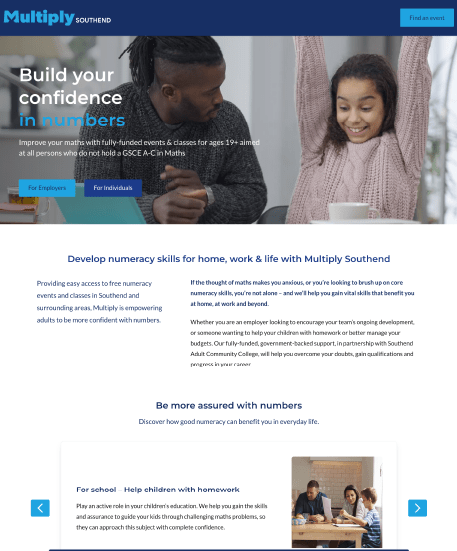**Caption:**

This promotional image for "Multiply South End" features a family engaged in a collaborative learning environment. The top section of the image has a dark blue bar with the text "Build your confidence in numbers, improve your math," highlighting the program's aim to offer fully funded events and classes for individuals aged 19 and above who do not hold a GSE A through C in math.

In the top left corner, the word "Multiply" is prominently displayed, reinforcing the program's brand. Below, on the south end of the image, there is a light blue rectangle labeled "Find an event," which guides viewers on where to discover available math classes and community events.

The central portion of the image showcases a typical scene from one of these events: people working together on math problems. One person is wearing a black sweater, while another in a pink sweater enthusiastically raises her arm, cheering.

Supporting text emphasizes the wide-ranging benefits of the program. It promises to develop numeracy skills for homework and daily life, providing accessible and free numeracy events and classes in the South End area. The initiative is described as empowering adults to become more confident with numbers, offering support whether you're anxious about math, looking to brush up on core skills, or aiming to help with your children's education.

Whether you're an employer seeking to enhance your team's development or an individual who wants to better manage budgets and household finances, the program's fully funded, government-backed support structures, including apprenticeships in the South End and collaborations with 12 community colleges, are designed to help overcome numerical challenges.

The image is completed with a message that highlights the value of numeracy in daily life, especially for supporting children's education. It encourages adults to gain skills that can help them confidently guide their kids through challenging math problems, ensuring they can actively participate in their children's learning journey.

At the bottom right, there's a blue square with an arrow, reinforcing the call to action and directing viewers to find further information.